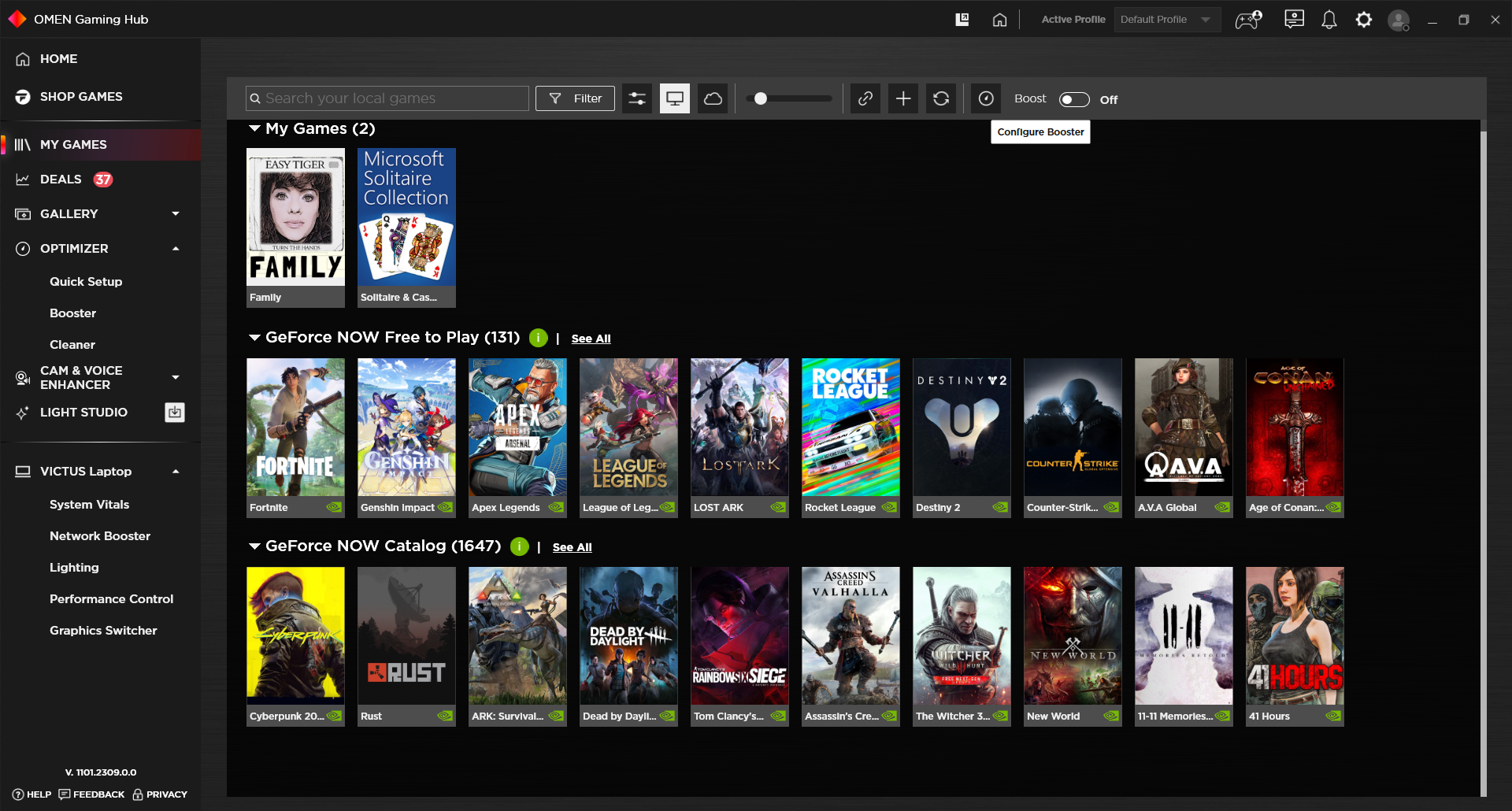In this detailed screenshot of the Omen Gaming Hub interface, the left sidebar features an extensive list of tabs including Home, Shop Games, My Games, Deals, Gallery, Optimizer, Quick Setup, Booster, Cleaner, Camera, Voice Enhancer, Light Studio, Victus Laptop, System Vitals, Network Booster, Lighting, Performance Control, and Graphics Switchers. 

On the main display, we are presented with a selection of games. At the top of the game list, there is an image featuring a girl with the title "Family" prominently displayed. Following this, the next game shown is Microsoft Solitaire Collection. Further down, we see a variety of popular games including Fortnite, Genshin Impact, Apex Legends, League of Legends, Lost Ark, Rocket League, Destiny 2, Counter-Strike, Ava, and Rust. The games are organized into three rows, with the first row featuring two games and the subsequent two rows each showcasing ten games. 

This comprehensive view highlights the versatility and breadth of options available within the Omen Gaming Hub, catering to a wide range of gaming preferences and system optimizations.